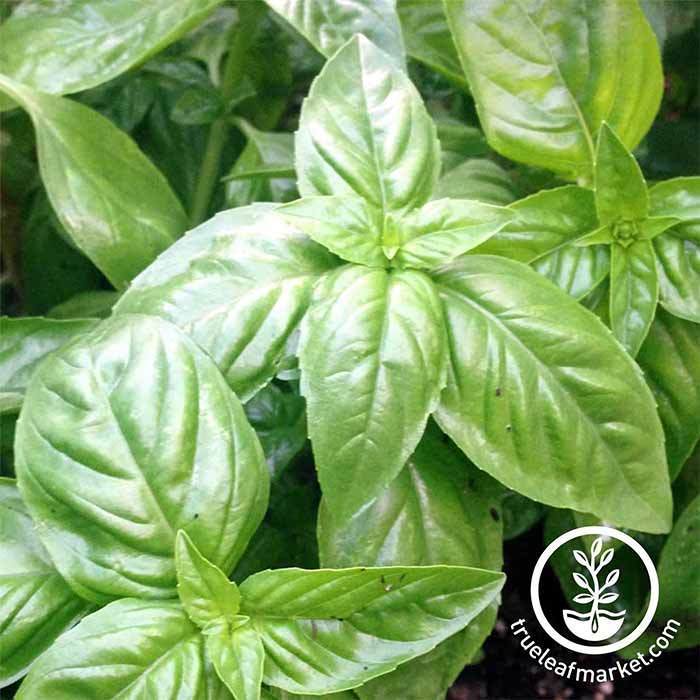The zoomed-in photograph captures multiple green leaves from what appears to be the same kind of plant, possibly basil. The leaves are large, oval or teardrop-shaped with pronounced veins and soft-looking spikes along the edges. They are arranged in a pattern where the smaller leaves are at the top, gradually increasing in size towards the bottom. The leaves are thriving uniformly without any flowers among them. Noteworthy are a few black spots visible on some of the leaves, particularly on a middle plant and one leaf at the bottom.

The background shows the brown soil from which the plant grows, speckled with white or gray remnants of dead vegetation or other detritus. Dominating the bottom right corner of the image is a logo overlaid on the photograph. This logo consists of a white circle with a sprout inside it, accompanied below by the text "trueleafmarket.com" in white.